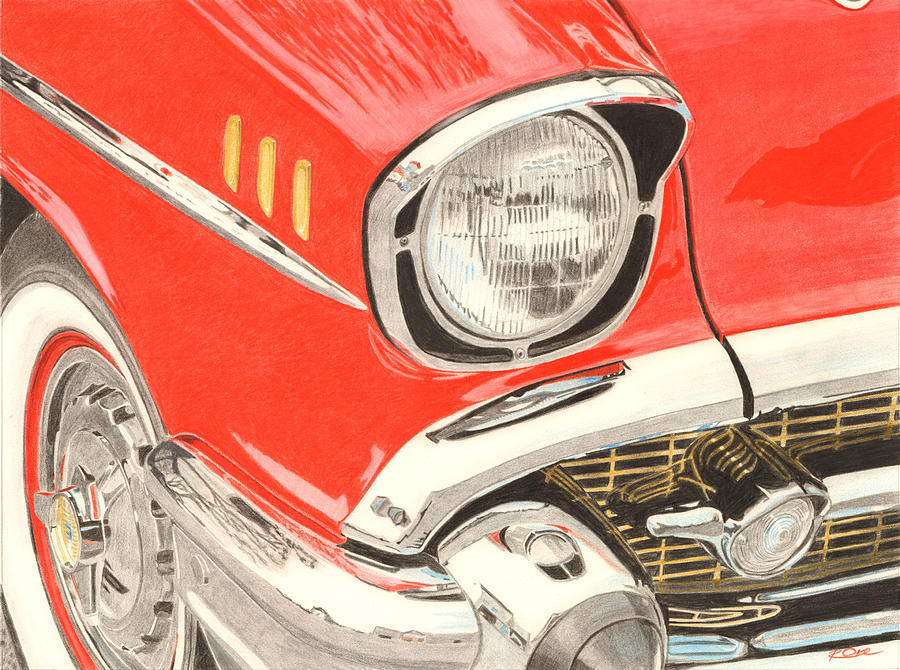This detailed image captures the front portion of a classic red car, focusing on distinct elements such as the front right wheel, partial front fender, headlight, and grille. The car, with its sleek and rounded design, features a prominent circular headlight accented by a small hood. Around the headlight, there are three smaller yellow blinkers positioned to the left. The grille, gold-colored and adorned with smaller lights, is flanked by polished chrome accents that extend along the bumper, fender, and sides. The wheel boasts a white wall with a red center surrounding the chrome hubcap, harmonizing with the car’s overall color scheme of red and silver. The classic vehicle’s highly polished chrome trims and rounded shapes emphasize its vintage and elegant style.